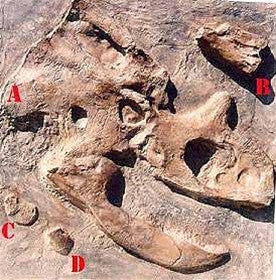The photograph, square-shaped and measuring approximately 1.5 to 2 inches on each side, captures a fossil partially excavated from a rock formation, likely by archaeologists, during daytime. The fossil display is meticulously labeled with large, bold red letters identifying four distinct parts. Situated on the upper left, marked as A, is a section that may be part of a skull or hip bone, somewhat resembling a horned cartoon face with an open mouth facing right. On the right side of the photograph, labeled B, lies a separate broken-off piece that resembles a horn. In the lower left-hand corner, two objects are labeled: a bean-shaped item marked C above a rounded object marked D. The surrounding rock is a mix of brown and gray hues, blending with the brown fossil, making the identification intricate yet detailed.